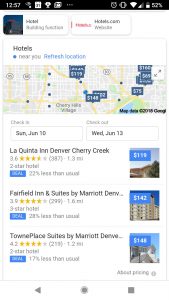This screenshot captures a somewhat blurry image displaying a Google Maps search for hotels. The screenshot itself is of low quality, making some text difficult to read. 

At the very top, the header is black with the time displayed on the left as 7:57. On the right, the battery indicator shows a 52% charge. Additional icons include Wi-Fi, wireless connection, an active alarm, and a mute indicator. 

Directly beneath the header, there appears to be an advertisement for hotels.com, featuring the site's name in what seems to be a repetitive manner; however, the text is quite indistinct. 

Below the ad, the Google Maps interface shows a segment titled "Hotels" but the map details remain unclear due to the blurriness. Rectangles indicating prices are visible albeit unreadable. 

Further down, the check-in and check-out dates are displayed as Sunday, January 10th, and Wednesday, January 12th, respectively. The first hotel listing is for La Quinta Inn, Denver Cherry Creek, which shows a 3.6-star rating. A photo accompanies this listing, but it is very pixelated. The price appears in a white font on a blue background and seems to be $159, though it's not entirely clear. 

The second hotel listed is the Fairfield Inn and Suites by Marriott Denver, with a 3.9-star rating and a more legible price of $142. 

Finally, the last listing shown is the Tower Place Suites by Marriott Denver, which has a 4.2-star rating. The price appears to start with $140 but the last digit is ambiguous, potentially being a 6 or an 8. Despite the blurriness, these key details can be distinguished.